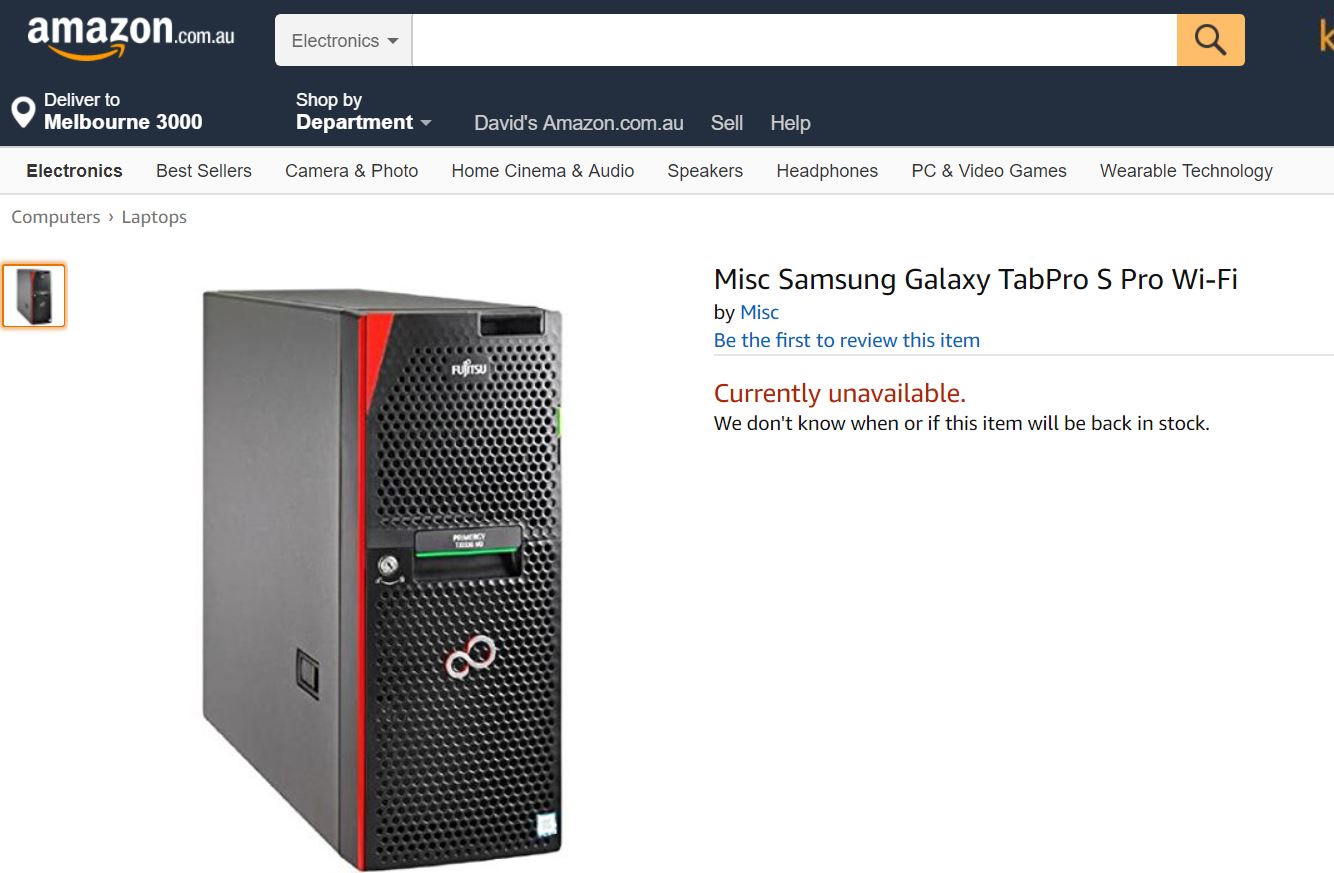In this image, we are observing an Amazon listing on the Australian Amazon website, davidsamazon.com.au. The top section of the image features a black background with the Amazon logo positioned on the top left. Adjacent to the logo is a white search bar, beside which lies an orange square housing a magnifying glass icon.

Just beneath the search bar, on the left-hand side, a gray text announces, "Deliver to Melbourne 3000." This is followed by navigation options listed as "Shop by Department," “Sell,” and "Help."

Directly below, eight categories of products are lined up from left to right. These categories include: Electronics, Bestsellers, Camera & Photo, Home Cinema & Audio, Speakers, Headphones, PC & Video Games, and Wearable Technology.

Further down, the main section of the image displays a specific product: the Samsung Galaxy Tab Pro S Pro Wi-Fi by MISC. This item is currently labeled with a blue text prompt, "Be the first to review this item," followed by a red alert indicating its status as "Currently unavailable." A message below clarifies that the restock date is uncertain.

On the left side of the product description is an image of the Samsung Galaxy Tab Pro S Pro Wi-Fi. The front surface of the device is black and designed with multiple holes, presumably for ventilation. The sides and top of the device are gray, and a striking bright red stripe runs vertically along the left-hand side of the product's front.

This elaborate layout and detailed product description not only highlight the device but also enhance the user's browsing experience on the Amazon platform.